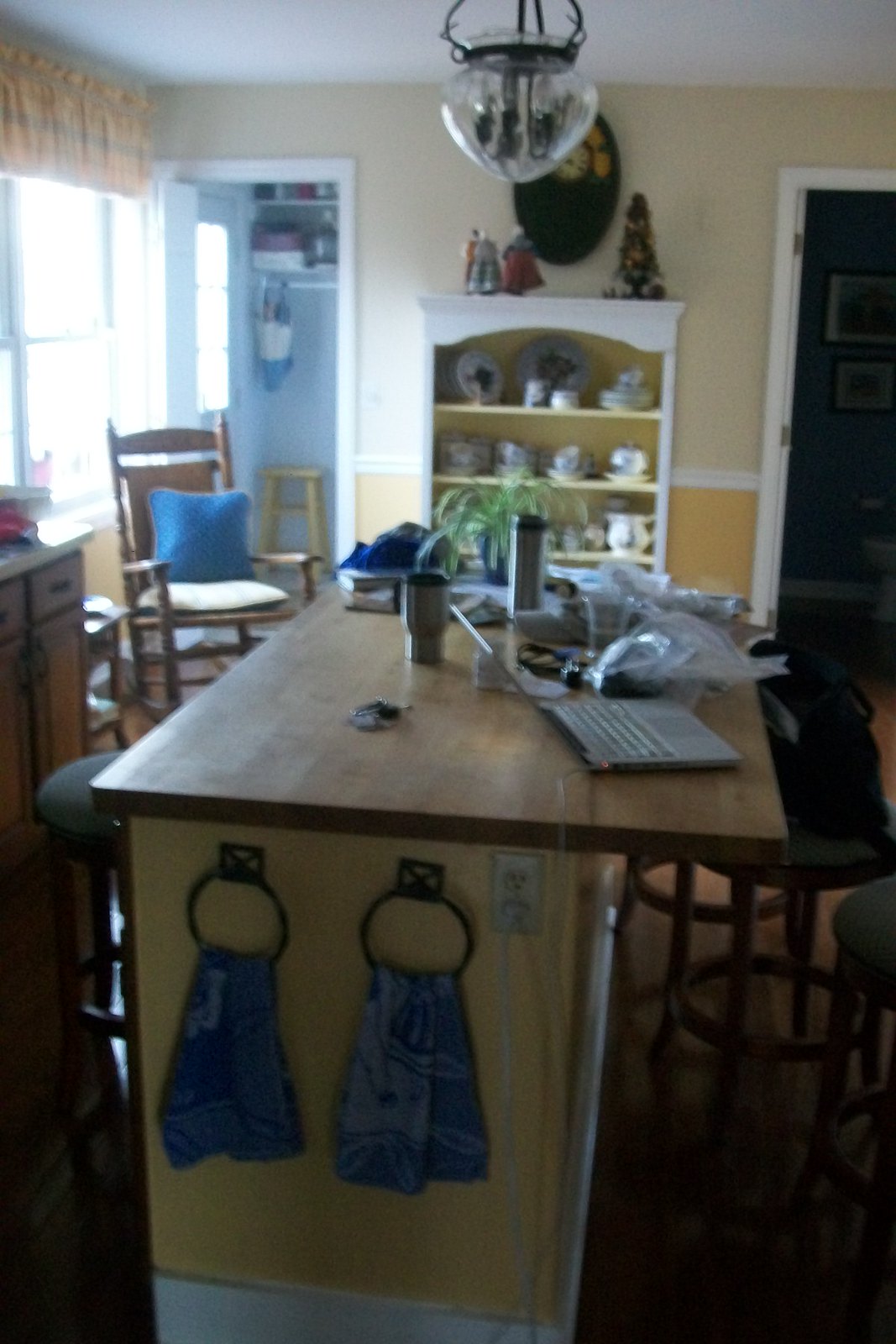A slightly out-of-focus and poorly lit color photograph captures the essence of a lived-in kitchen. The perspective looks along an eat-in bar, showcasing kitchen cabinets to the left, which are barely visible. A wood-topped counter functions as a bar, adorned with stools. At the end of this bar, two towel rings hold towels, and nearby, an electrical outlet powers an open laptop resting on the bar. Next to the laptop, there is an insulated travel thermos-style cup. Plastic bags clutter the countertop, while a backpack or purse sits on one of the stools.

Further down the bar, a decorative bookshelf, painted and shaped with an arched top, displays fine china rather than books, effectively serving as a china cabinet. A clear glass, bowl-shaped light fixture hangs above the bar, illuminating the scene dimly. A bright window on the upper left side of the photo is adorned with a puffy valance curtain, allowing natural light to spill in. The walls are painted a light yellow on the upper half and a richer, orangey yellow on the lower half, all trimmed in white.

Through a narrow doorway on the left, a glimpse into what appears to be a pantry reveals shelving and a stool. Below the window, a cane and wood rocking chair with a blue back cushion adds a touch of homeyness. Another darker doorway on the right leads into what could be a hallway or another room, featuring framed art on the walls.